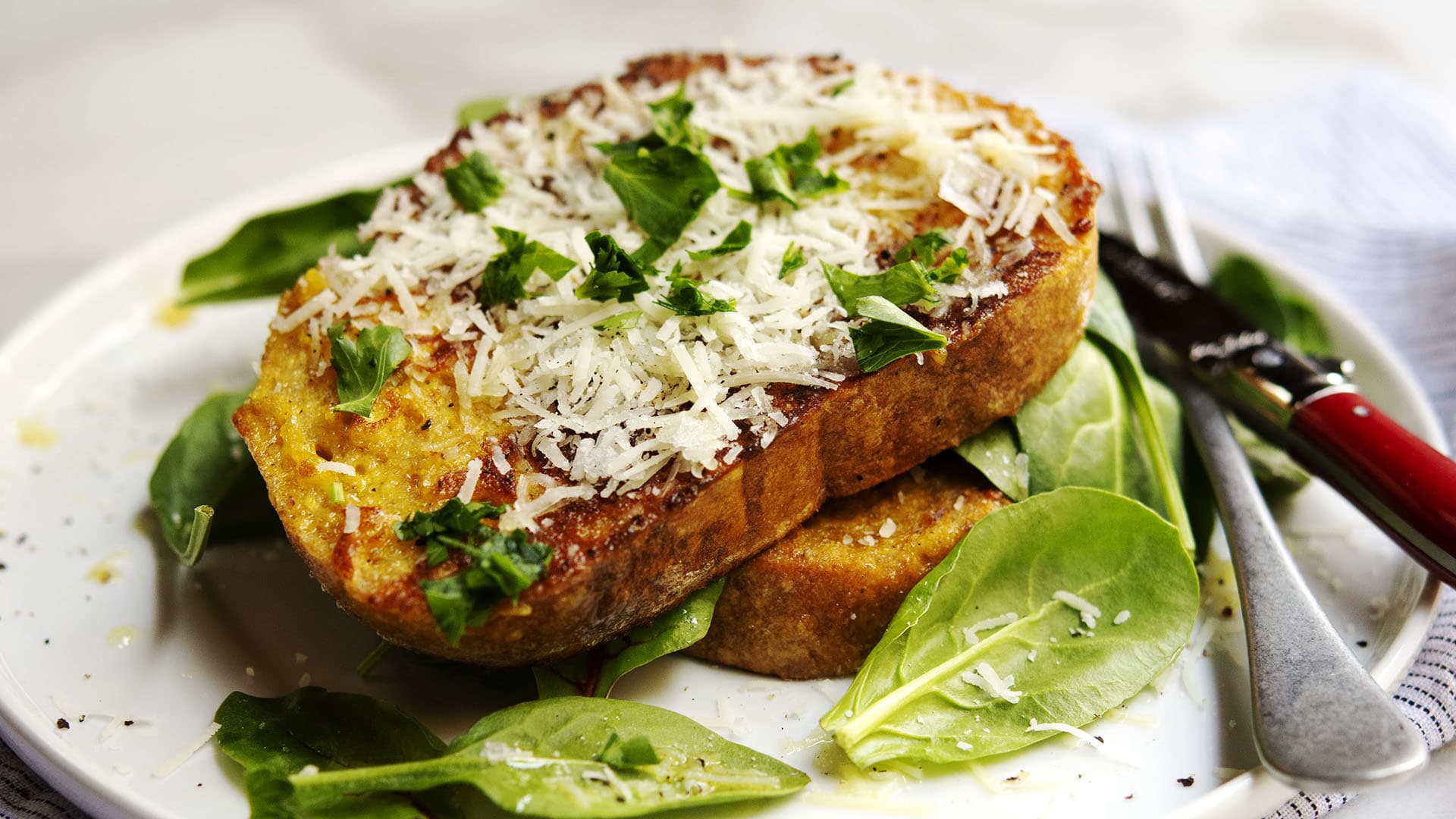This is a photograph of a white, circular plate set on a white tablecloth with black dotted stripes. The plate features a neatly arranged meal consisting of two pieces of garlic toast, one almost completely obscured by the other. Each toast is egg-battered, fried, and generously topped with shredded white cheese and finely chopped greenery, likely parsley. Scattered around the toast is a bed of fresh spinach. A chrome fork is placed on the right-hand side of the plate, while a knife with a red (or mahogany) handle lies alongside it, with their positions slightly crossed. The detailed setting and delicious toppings create an inviting scene, ready to be enjoyed.